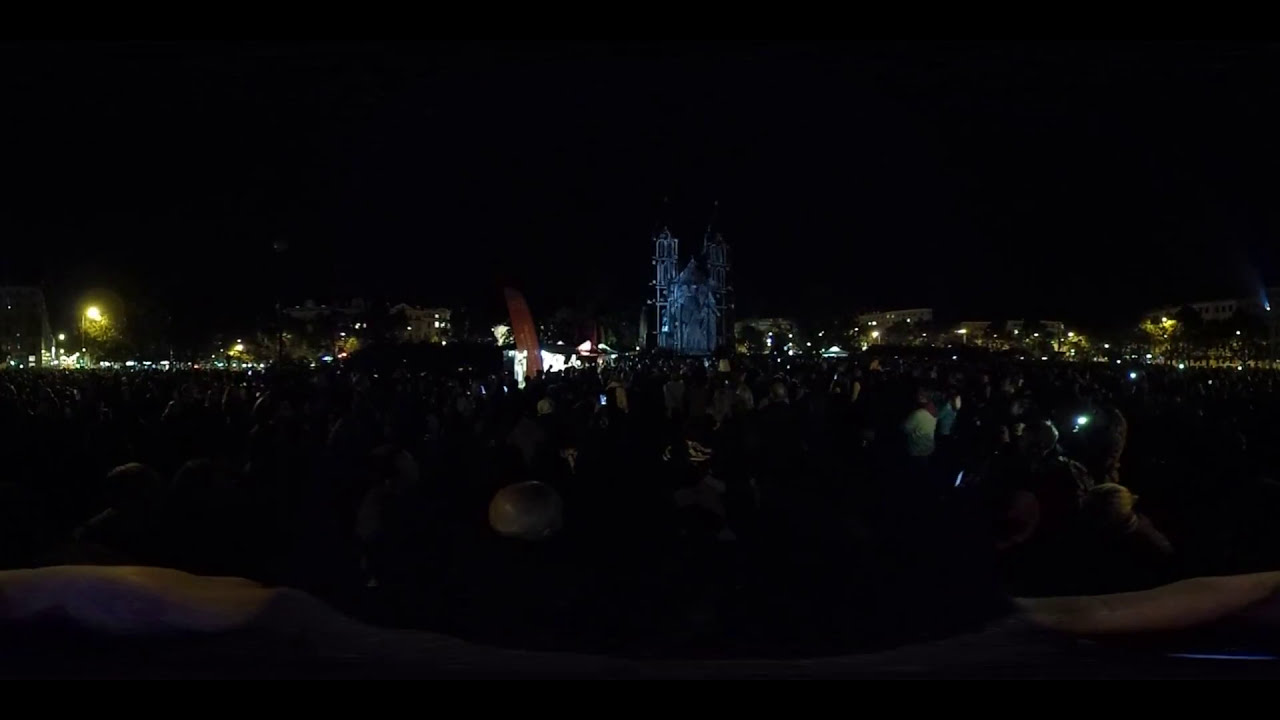The image captures a nighttime scene with an atmospheric cityscape in the background featuring numerous illuminated buildings and trees. In the foreground, a large crowd of people is gathered, many holding up cell phones, suggesting the setting might be a concert or festival. These individuals appear to be standing on what resembles a boat or raft, due to a brown object extending horizontally at the bottom of the frame. Dominating the center of the image is a striking, gray-blue building with a distinct architectural style reminiscent of a church, complete with two large towers on the left and one on the right. The dark sky overhead and the subtle lights scattered throughout the scene further enhance the nocturnal ambiance.